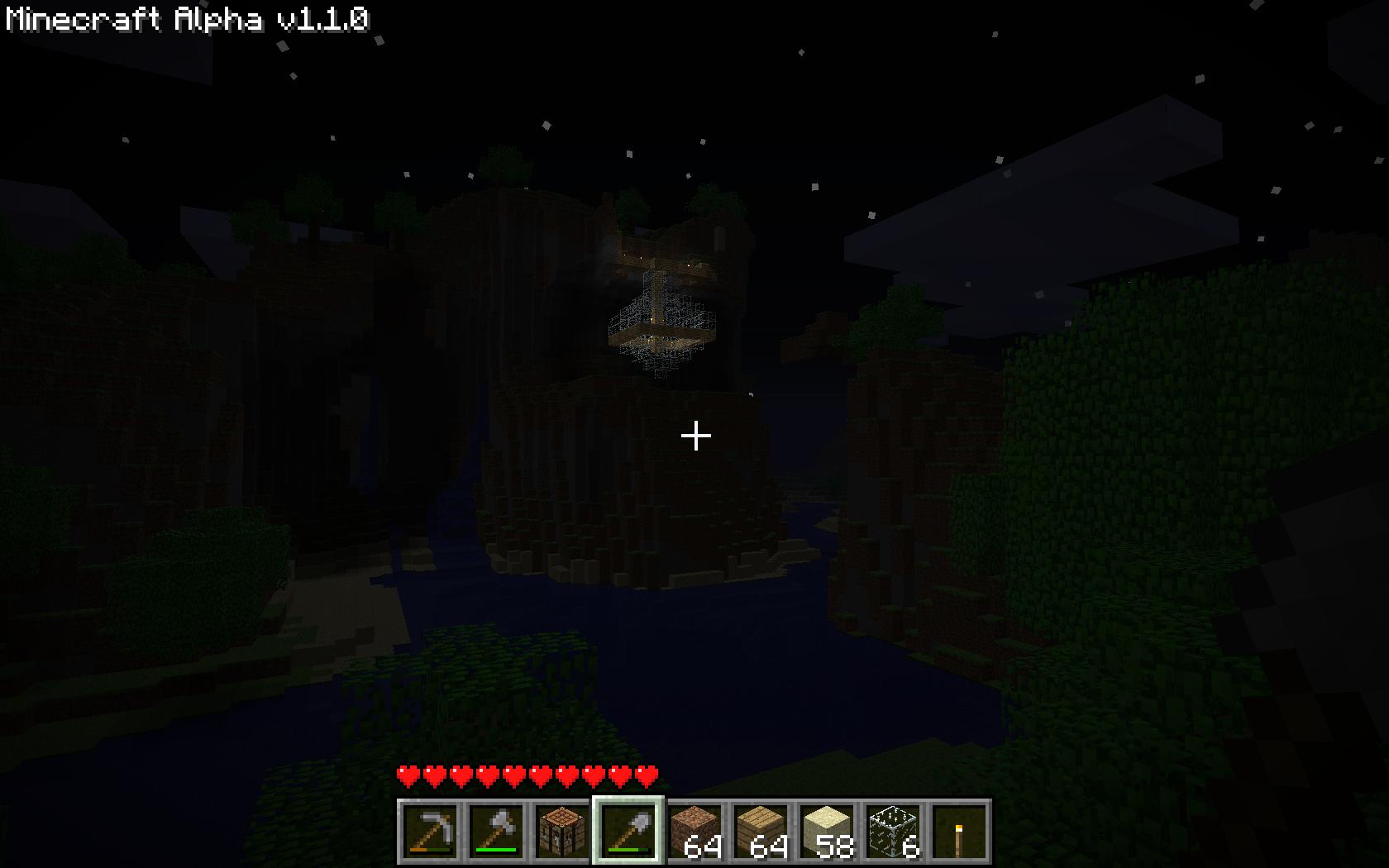This image appears to be a screenshot from the video game "Minecraft Alpha," version 1.1.0. The screen is predominantly black, evoking the vastness of space, with tiny white specks dotting the upper portion, resembling stars. Central to the image is a brown and gold object, possibly a small figurine or a helicopter-like structure. Below this object is a white cross, comprised of a vertical and a horizontal line.

At the bottom of the screen, a row of 10 small boxes is displayed, each likely representing the player's inventory slots. Above these boxes, there are 10 red hearts, indicating the player's health status. The first inventory slot contains a tool resembling a sword, while the second slot holds an object that looks like a hammer. The subsequent slots contain a box, a spatula-like tool, another box, and four differently colored boxes: brown, light brown, off-white, and one that is black with white specks. The final slot contains a gold bar. Numerical values above the colored boxes indicate quantities: 64, 64, 58, and 6.

In the background, faint details are visible against the black, although they are not clearly discernible. At the top of the image, the text "Minecraft Alpha V1.1.0" is displayed in white.